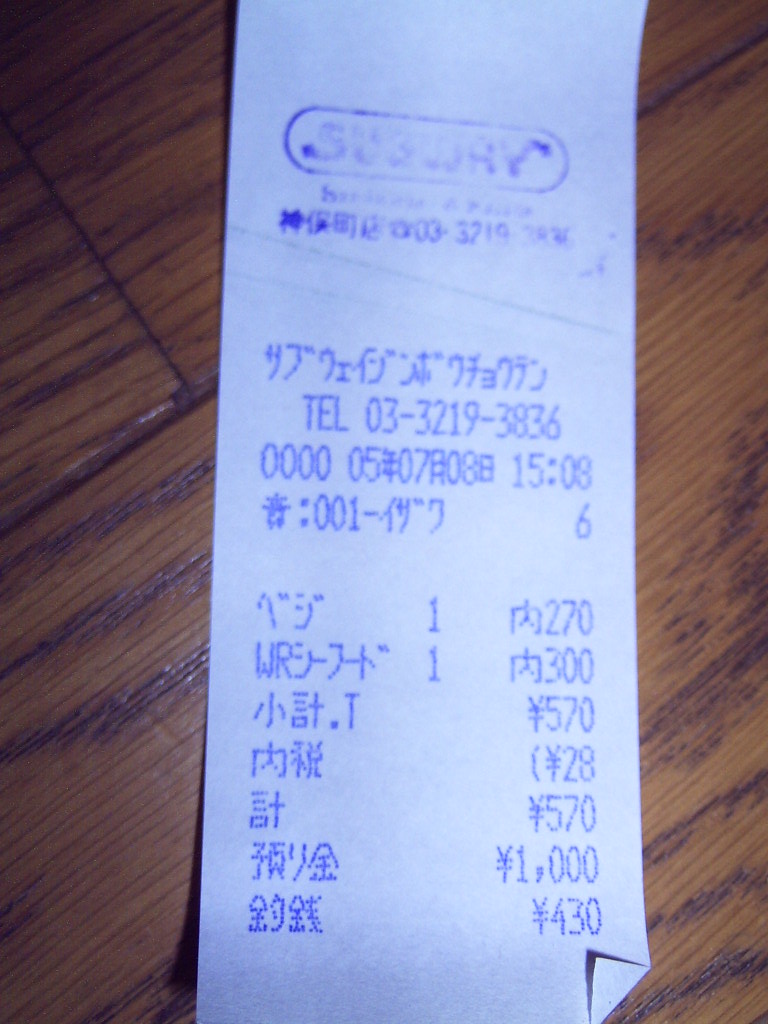This photo captures a detailed close-up of a Subway restaurant receipt from what appears to be Japan, evidenced by the presence of Japanese characters and yen symbols. The receipt rests on a beautifully grained wooden surface, potentially a table or floor, with visible joints that give it a slightly rustic appearance.

At the top of the receipt, the familiar Subway logo and name are printed in bluish ink. Just below the logo, there's additional text which could be an address or contact information in Japanese, followed by a clearly visible phone number in English: 03-3219-3836. 

The receipt also includes a store number and the time of the order, indicated as 1508. Listed beneath are several items along with their corresponding prices: 270 yen, 300 yen, 570 yen, 28 yen, 570 yen, 1000 yen, and 430 yen, which likely represents the total change given to the customer.

A small detail at the bottom right-hand corner of the receipt shows it slightly folded up, adding a touch of casual authenticity to the image. This meticulously detailed composition provides a curious glimpse into an everyday transaction in an Asian country, specifically Japan.